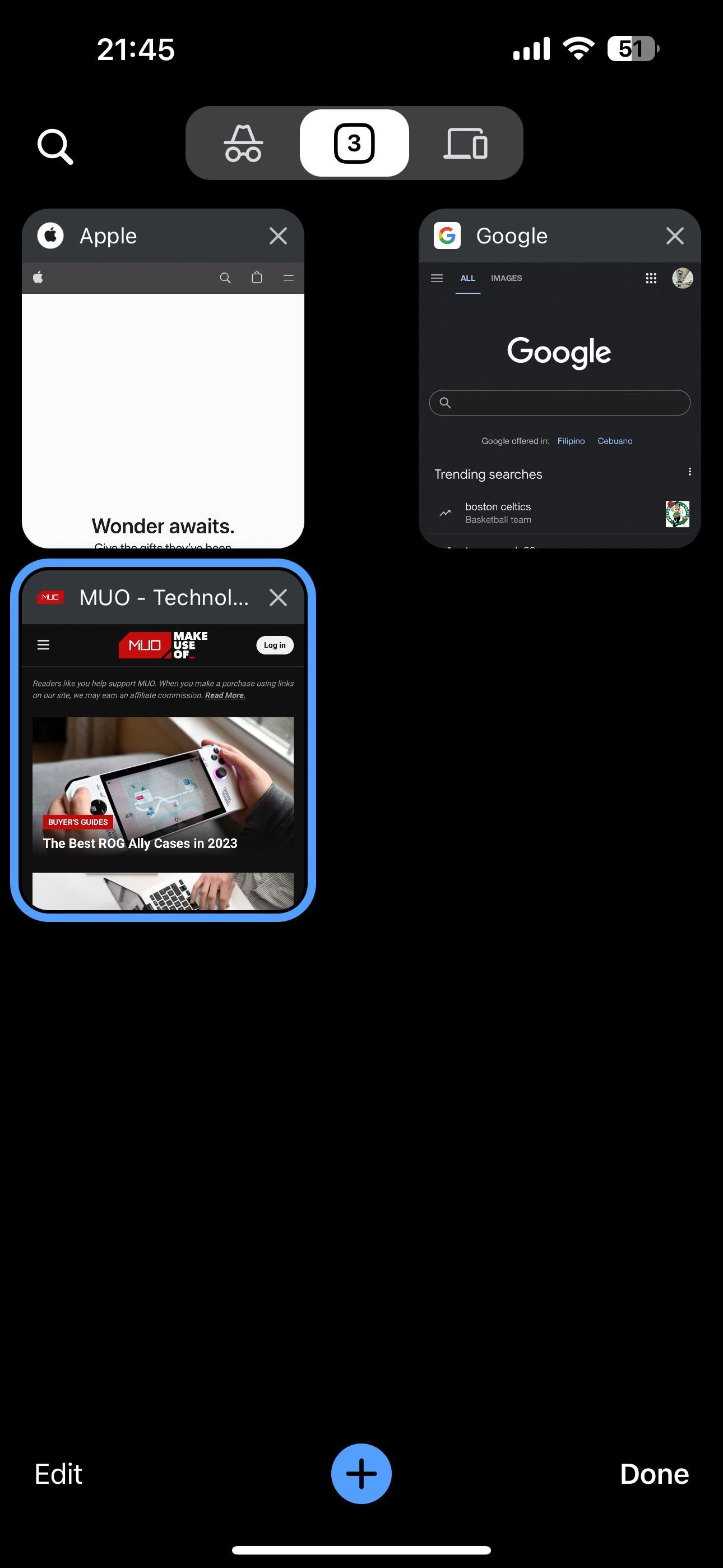A screenshot captured at 12:25 PM (military time) is displayed on a phone with a black background. The phone shows full signal bars, Wi-Fi is enabled, and the battery is at 51%. The screen is in an incognito mode, denoted by an icon of a hat with glasses, and features an option to switch between tablet and phone layouts. The screenshot appears to be from the tab management view, where the user is selecting from their open pages.

The first tab is an Apple page, which is mostly blank except for the text "Wonder Waits" at the bottom and a small bar across the page, resembling an Apple search or menu option. The second tab is a Google search page displaying trending searches, an "images" option, and the user's avatar on the right-hand side.

Currently, the highlighted tab with a blue outline is "MUO Technology," a site that reviews electronics, specifically showcasing "the best Rock Ally cases of 2023." At the bottom center of the screen is a blue circle with a black plus sign, indicating the option to open a new tab. On the left in white is the "Edit" option, and on the right in white is the "Done" option, suggesting the user is managing their open tabs.